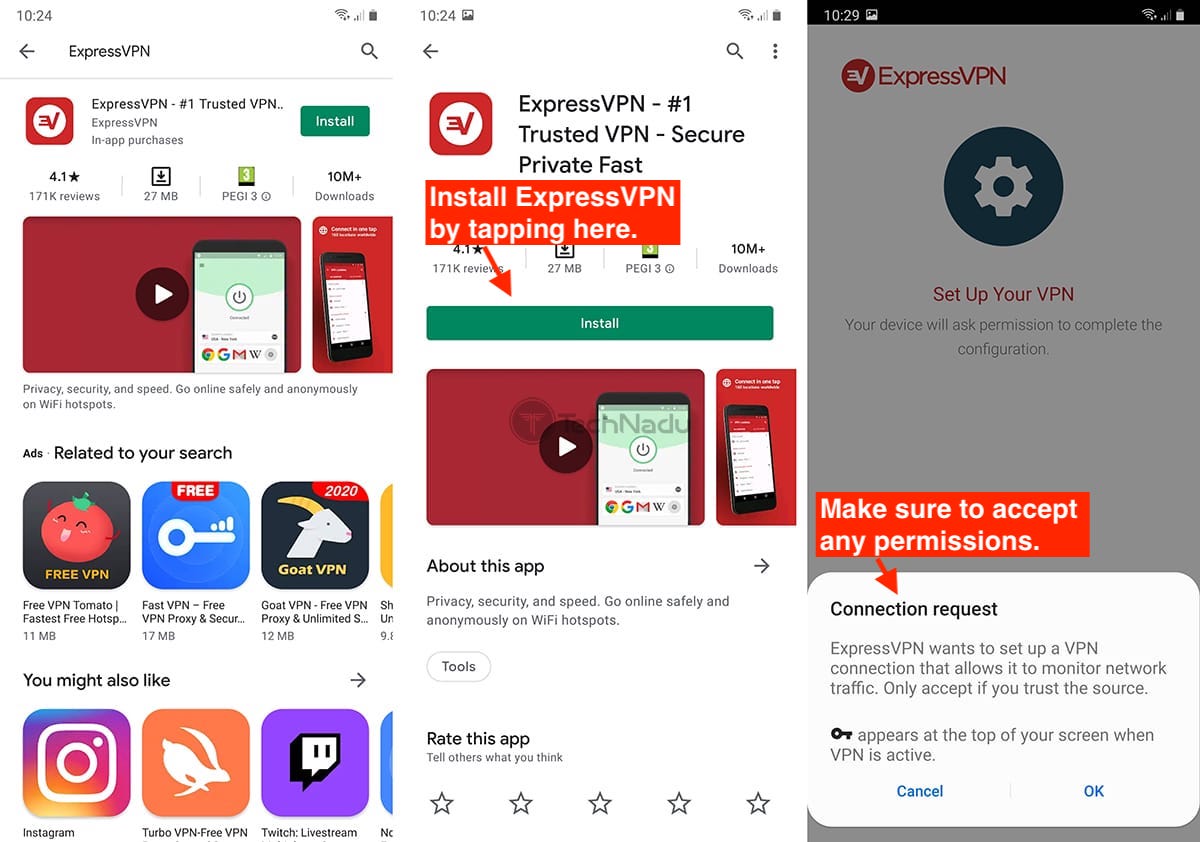Three vertical, side-by-side screenshots depict different stages of interacting with the Express VPN app on a mobile phone. Each image is timestamped at either 10:24 or 10:29, indicating that they were taken within a close time frame.

In the first screenshot, labeled 10:24, the Express VPN app is displayed as a search result in an app store. The layout features the app name, "Express VPN - #1 Trusted VPN," along with its red and white logo. At the top of the screen are typical phone status icons like battery level and Wi-Fi signal. Below the app title is an "Install" button, indicating that the app has not yet been downloaded. Underneath this section are recommendations for other apps and various advertisements, including logos for Instagram and additional suggested applications.

The second screenshot, also marked at 10:24, shows a detailed app page for Express VPN. This page is predominantly red and white, consistent with the app's branding. It includes a comprehensive description of the app's features, user ratings, and screenshots illustrating how the app functions. It appears to be the display seen after tapping on the app from the search results in the app store.

The final screenshot has a timestamp of 10:29. This image shows the app in action after installation, with a setup screen that prompts the user to configure their VPN settings. A central wheel graphic is displayed with instructions to "Set up your VPN" and additional guidelines about accepting permissions and connection requests to finalize the setup. 

All three screenshots collectively narrate the process of searching for, viewing, and setting up the Express VPN app on a mobile device.